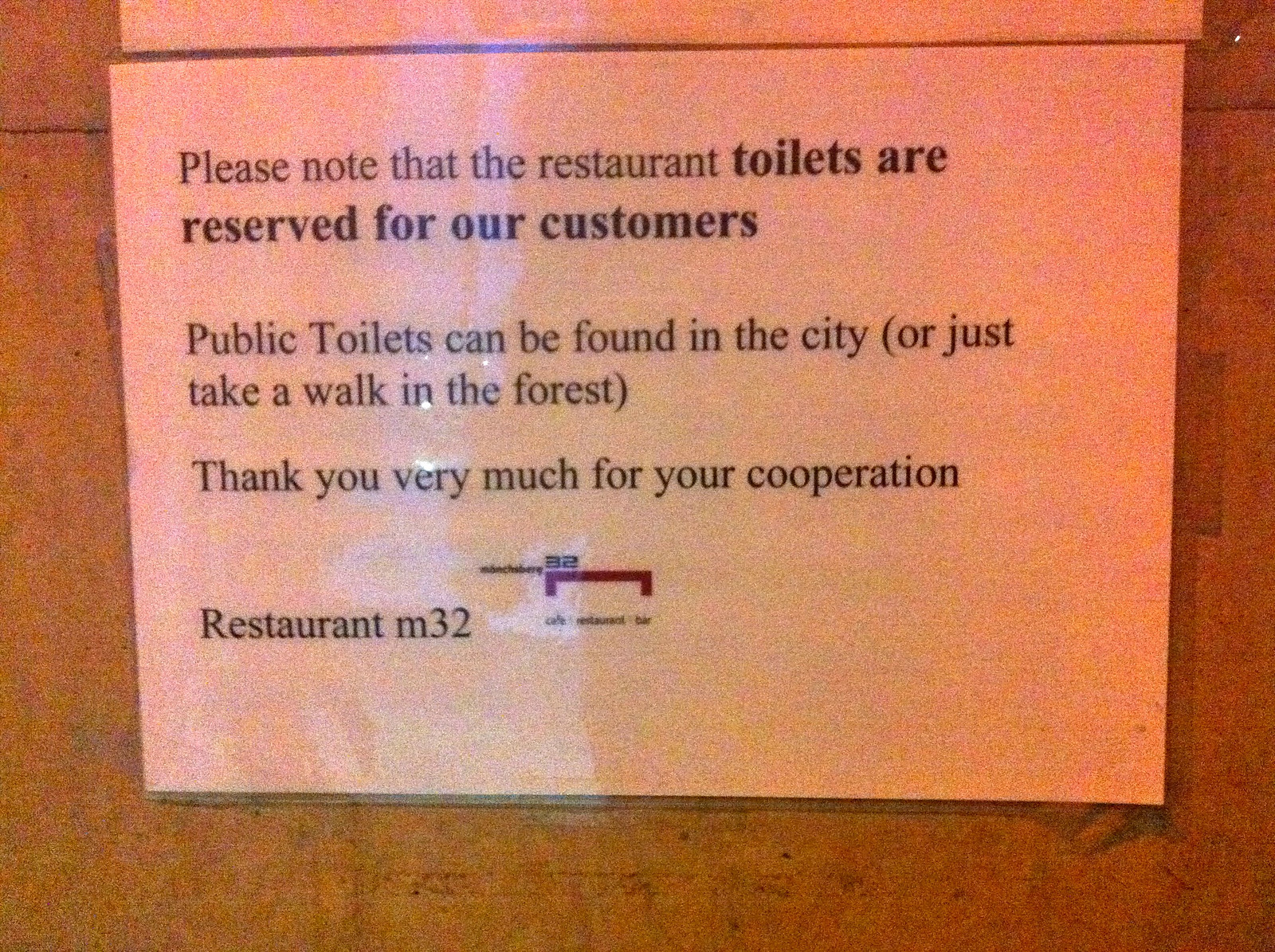In this photograph, a laminated sign is centrally affixed to a brown or tannish wall, likely in a restaurant setting near the restroom. The sign, which appears white with black and red text, states: "Please note that the restaurant toilets are reserved for our customers. Public toilets can be found in the city (or just take a walk in the forest). Thank you very much for your cooperation. Restaurant M32." The title "Toilets are reserved for our customers" is in bold for emphasis. A small, slightly obscured logo due to glare from the lamination appears alongside the text. The overall image has a warm, orange tint, likely influenced by the indoor lighting. The simplicity of the setup with no additional objects or text besides the sign enhances the focus on the message conveyed.